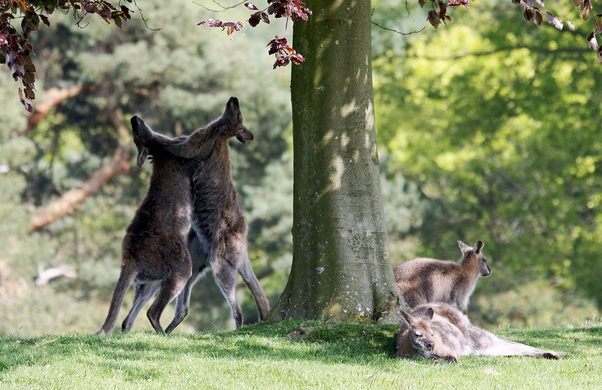The image captures a vibrant outdoor scene set on a warm summer day. At the center of the image is a large, thick tree with a trunk approximately two feet in diameter. The tree, adorned with dark red leaves, provides ample shade for the area around it. On the right-hand side of the tree, there is a kangaroo laying flat on the lush, neatly trimmed green lawn, while another kangaroo sits nearby, gazing into the distance. To the left of the trunk, two kangaroos are engaged in a playful or possibly antagonistic fight, standing on their hind legs with their heads tilted back, front legs pressed against each other as if boxing. The kangaroos have light brown, fuzzy fur coats, with white fur on their stomachs and inner legs. Their long, thick tails are clearly visible, and the insides of their ears display a pinkish hue. The background is filled with green trees and some branches, all nicely lit by sunlight, enhancing the overall serene yet dynamic atmosphere of the scene.